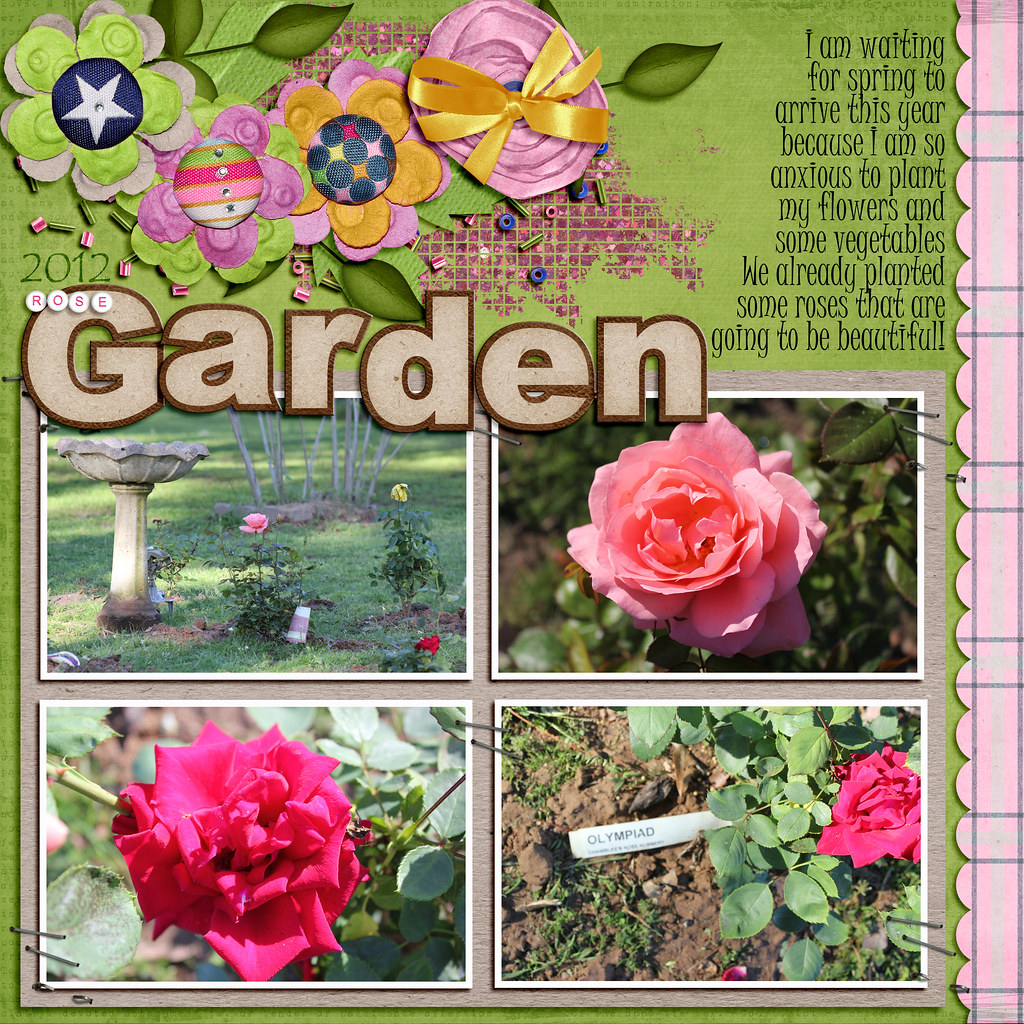This image shows the cover of a meticulously crafted scrapbook titled "2012 Rose Garden". The overall background of the cover is adorned in a pale olive green hue, accentuated by a light pink scalloped border on the right, featuring light gray and mint green pinstripes. Dominating the center, four carefully placed photographs of roses are showcased. In the upper left photo, four rose plants surround a birdbath amidst a grassy field, with vibrant pink and yellow roses in bloom. To its right, an up-close shot captures a delicate open pink rosebud. The lower left photograph displays a darker pink rosebud in full bloom, encased by lush green leaves, while the lower right features a similarly bloomed pink rose marked with a tag reading "Olympiad". The scrapbook cover is further embellished with hand-created designs of overlapping paper mache flowers and fabric roses, complete with ribbons and a subtle glitter finish. A text block at the upper right, penned in black, expresses, "I am waiting for spring to arrive this year because I am so anxious to plant my flowers and some vegetables. We already planted some roses that are going to be beautiful."